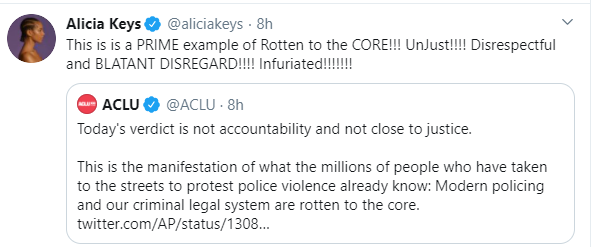[Image Caption]

The verdict delivered today starkly epitomizes the systemic issues entrenched in modern policing and the criminal legal system. This outcome, branded as excessive and disrespectful, falls disastrously short of true accountability and justice. The image represents the profound frustration and fury felt by millions who have protested against police violence. It underscores the pervasive sentiment that our justice system is fundamentally flawed and deeply unjust. The American Civil Liberties Union (ACLU) highlights this with their statement, reinforcing the notion that the current state of affairs is a blatant disregard for genuine justice. This exact sentiment is echoed across multiple platforms, as seen on Twitter, where users unite in their condemnation of such failures in our legal system.

#Policing #Justice #ACLU #Protest #SystemicIssues #PoliceViolence

(Note: Verification details such as "ACLU, 8 hours" and "electric keys, 8 hours" were not included as they seem extraneous to the main message of the caption.)